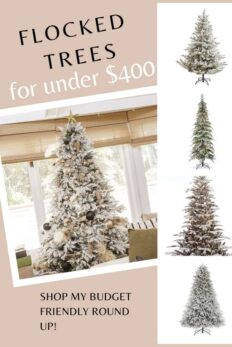The image resembles a pamphlet or a homepage for a website dedicated to flocked Christmas trees. 

On the left, there's a tan section featuring a Christmas tree positioned in what appears to be a sunroom, basking in natural light. At the top of this section, the text reads, "Flocked Trees for Under $400." Below the photo, an enthusiastic caption states, "Shot my budget from the round up!"

To the right is a white section showcasing images of four different flocked Christmas trees, each standing on a cross-shaped leg base. These trees, covered in white flocking to simulate snow, vary in style and shape:

1. The top tree is traditional, with branches (pines) facing up and mounted on a stand.
2. The second tree is thin, with its pines curling downward.
3. The third tree has a classic Christmas tree silhouette, broader at the bottom with slightly drooping pines.
4. The bottom tree has a rounded, almost pizza-like shape with dense white flocking, also on a base.

This section reiterates the theme with the caption, "Flocked Trees for Under $400."